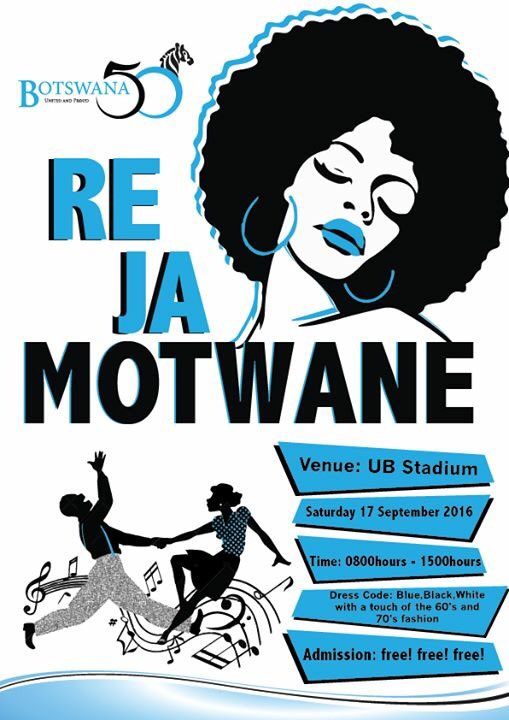This vibrant concert poster, set against a clean white background with black and light blue accents, prominently features the celebration of "Botswana 50" in the top left corner. The central title, "Re Ja Motwane," is bold and striking, drawing attention to the event’s name. Dominating the top right of the poster is a captivating pop-art styled image of an African American woman with a large black afro, closed eyes, and blue lipstick, adorned with prominent blue hoop earrings, her head tilted thoughtfully to one side.

Further details are vividly illustrated at the bottom of the poster. On the bottom left, lively graphics depict two African American figures dancing amid musical notes, emphasizing the event's festive atmosphere. The bottom right corner provides essential information: the venue is UB Stadium, the date is Saturday, September 17, 2016, from 8:00 AM to 3:00 PM, with a dress code that suggests wearing blue, black, or white with a 60s and 70s fashion twist. Admission to the event is proudly noted as free, making it an accessible celebration for all.